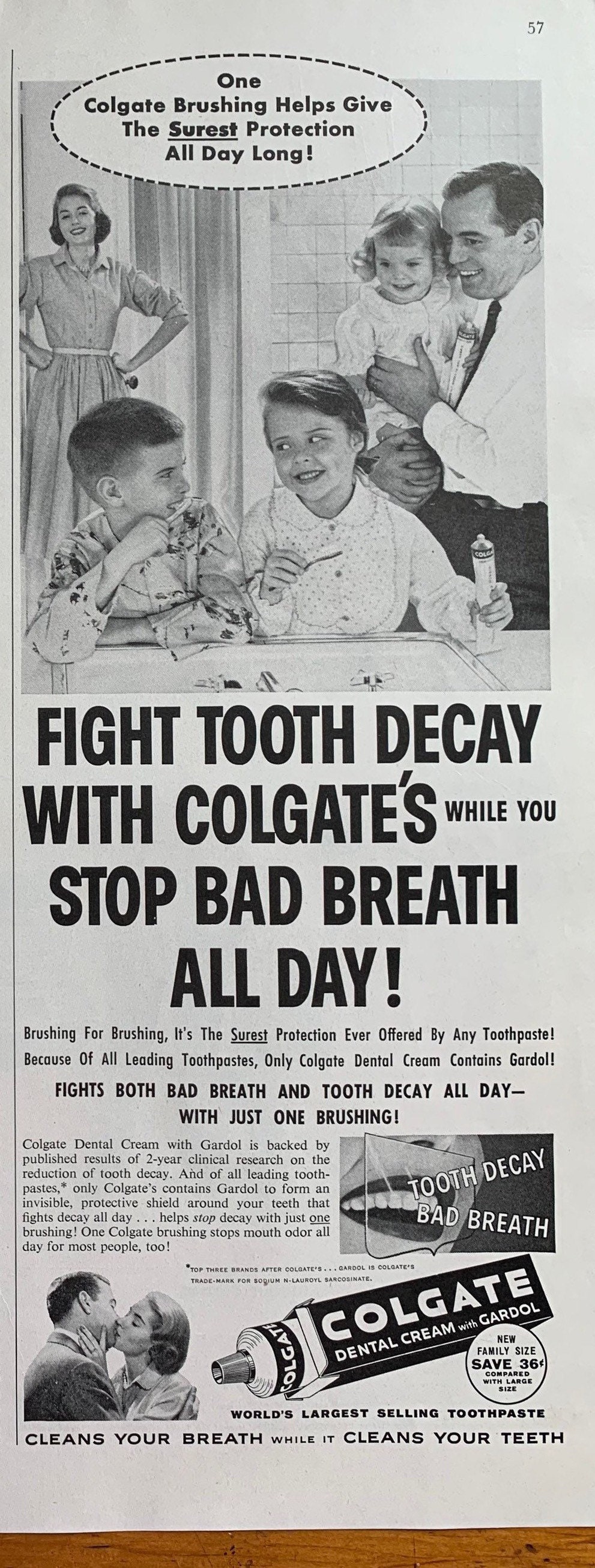This vintage advertisement from the mid-1950s for Colgate toothpaste is presented in a black-and-white newspaper format, possibly lying on a wooden table, adding a nostalgic touch to the scene. The ad is structured as a long vertical rectangle filled with engaging details. At the top, bold black font exclaims, "One Colgate brushing helps give the surest protection all day long!" Below this headline, a black-and-white photograph features a cheerful family: a mother, father, and their three children. The father holds a young girl in his arms while a boy and another girl stand at a sink, brushing their teeth and smiling at each other. The mother, styled like a classic 1950s housewife with short hair and a long, full-skirted dress, smiles warmly from nearby. 

Below the family photograph, bold all-caps text commands, "FIGHT TOOTH DECAY WITH COLGATE WHILE YOU STOP BAD BREATH ALL DAY." A smaller paragraph underneath elaborates, "Brushing for brushing, it's the surest protection ever offered by any toothpaste. Because of all leading toothpaste, only Colgate Dental Cream contains Gardol. Fights both bad breath and tooth decay all day with just one brushing." 

The bottom section of the advertisement features additional visuals. On the left, a close-up of a woman's smiling mouth emphasizes the promise of fresh breath. Beside it, a romantic image of a couple kissing underscores the confidence provided by Colgate. Finally, a drawing of a Colgate toothpaste tube in its packaging closes the ad, reiterating its dual action: "Cleanse your breath while it cleans your teeth."